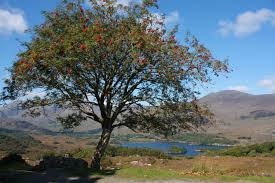In this small, horizontally rectangular image, we see a beautifully detailed scene captured during the daytime. In the foreground stands a thick tree, robust with green leaves and scattered with red flowers or possibly fruit. The tree's blackish trunk diagonally ascends to the right before branching out in several directions, creating a lush canopy that casts a shadow towards the left bottom part of the image.

Beneath the tree stretches a carpet of green grass, interspersed with patches of brown, possibly indicating sparse areas without grass. In the mid-ground, a serene lake or large pond with dark blue waters lies nestled, adding a sense of tranquility. Beyond the lake, rolling hills rise with a mix of rocky and grassy terrain, in hues of green and brown. The sky above is a vibrant blue, dotted with white clouds, completing the picturesque landscape. Far in the distance, a misty mountain range looms, blending harmoniously with the serene environment, evoking a sense of peaceful isolation away from urban life.